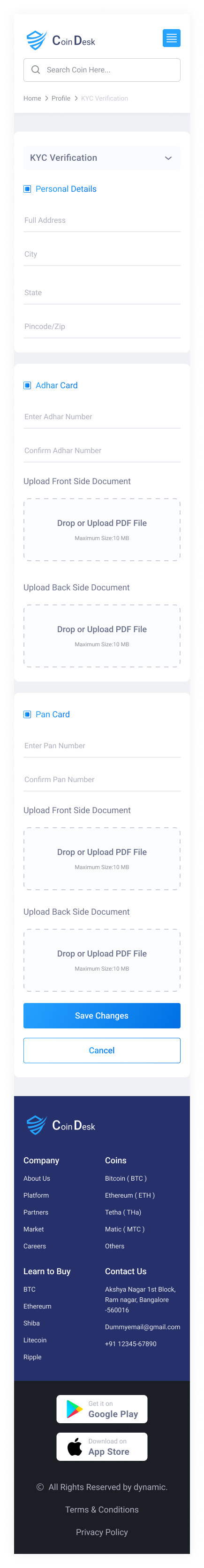This vertically-oriented portrait-style image appears to be a screenshot taken on a mobile phone, although it is notably squished, blurry, and difficult to read. The image represents the settings section of an application, potentially related to cryptocurrency, featuring a distinctive blue icon that might say "coin" something. 

The layout includes various elements typically found in settings menus: search fields, informational fields to fill out, and areas designated for uploads indicated by dotted lines. There are also "Confirm" and "Cancel" buttons, enhancing the interactive options available to users. 

At the very bottom of the image, copyright information and navigation options are faintly visible, along with download buttons for the Google Play Store and Apple App Store. Despite the intended clarity, the text and icons have become unreadable due to the vertical squish, distorting the image content. 

The background is predominantly white with black text, except for the section titles, which are highlighted in blue. It seems the screenshot was poorly executed, failing to properly capture the intended details of the application settings.